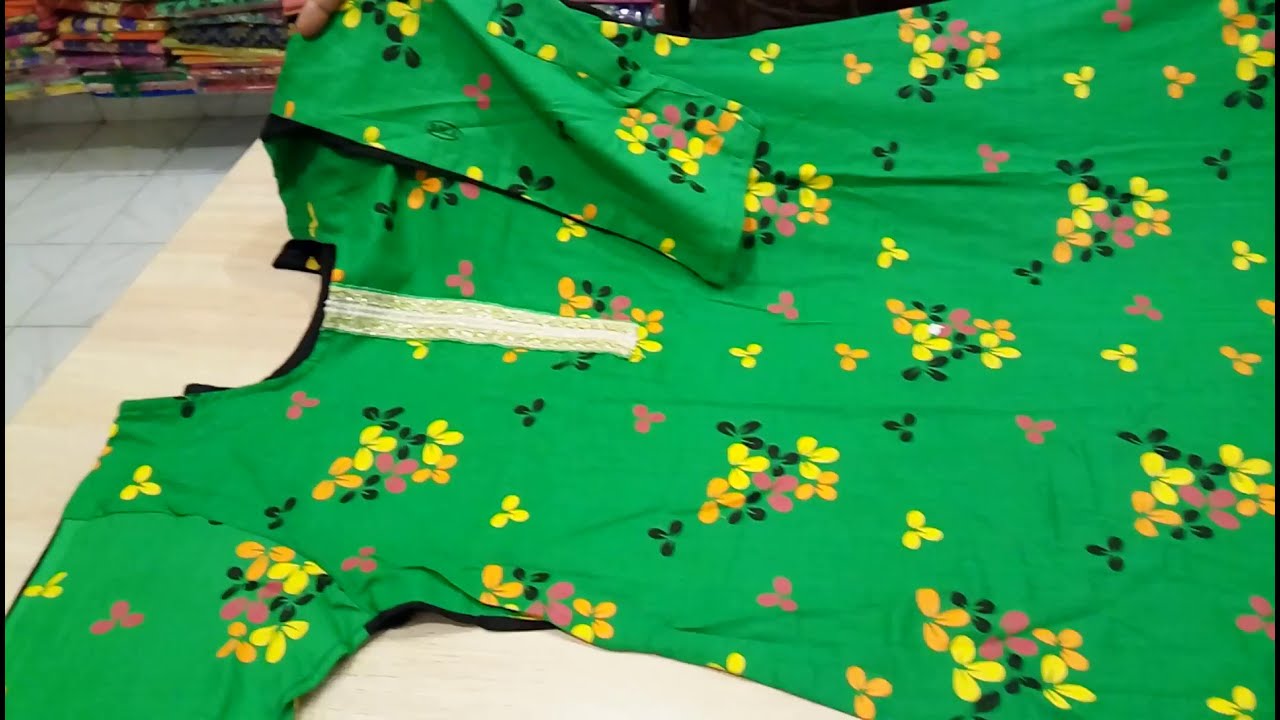This detailed color photograph, oriented in landscape, captures a vibrant green dress with short sleeves, adorned with floral prints in yellow, pink, orange, and black. The flowers, complete with green leaves, create an intricate and lively pattern. Central to the dress's design is a white lace strip running vertically from the neckline to the breast area, approximately six inches long. The dress lies on its side atop a light brown piece of muslin, which itself rests on a smooth, light wood table. The ground beneath the table features gray stone tiles, adding a contrasting texture to the scene. A person's fingers are visible, slightly lifting a corner of the sleeve, perhaps for closer inspection. Surrounding the main subject, the background includes a stack of colorful bolts of fabric, suggesting the setting might be a clothing or tailoring store. This realistic and detailed composition might be part of an instructional guide on garment construction.